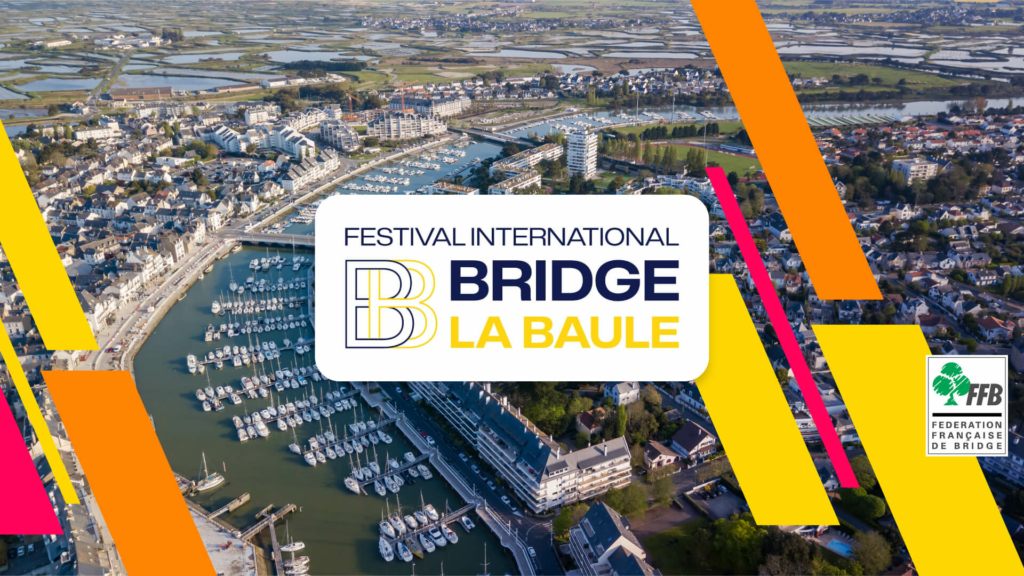This aerial photograph showcases a river winding through an industrial cityscape, bordered by buildings and docks filled with meticulously aligned small boats and yachts, resembling a marina. The river curves from the top right, arcing towards the left and returning towards the bottom, creating a dynamic flow through the scene. Overlaid on the image are prominent graphics and text. Centrally positioned is a white rectangular sign with rounded corners, displaying "Festival International" in black text on top. Beneath, two interlinked capital B's—one blue and one yellow—are set side by side. To the right of this, the words "Bridge" in dark blue, and "LA BAULE" in yellow capital letters appear. The design is accented with angular stripes in yellow, orange, and deep pink on the left, and additional stripes on the right in a descending sequence of orange, yellow, deep pink, and yellow. In the lower right corner is another white rectangular logo with "FFB" in blue, and below it, "Fédération Française de Bridge," indicating the French origin of this festival-themed imagery. The vibrant overlaid elements contrast with the industrial and aquatic tranquility of the underlying cityscape, creating a rich, layered visual narrative.